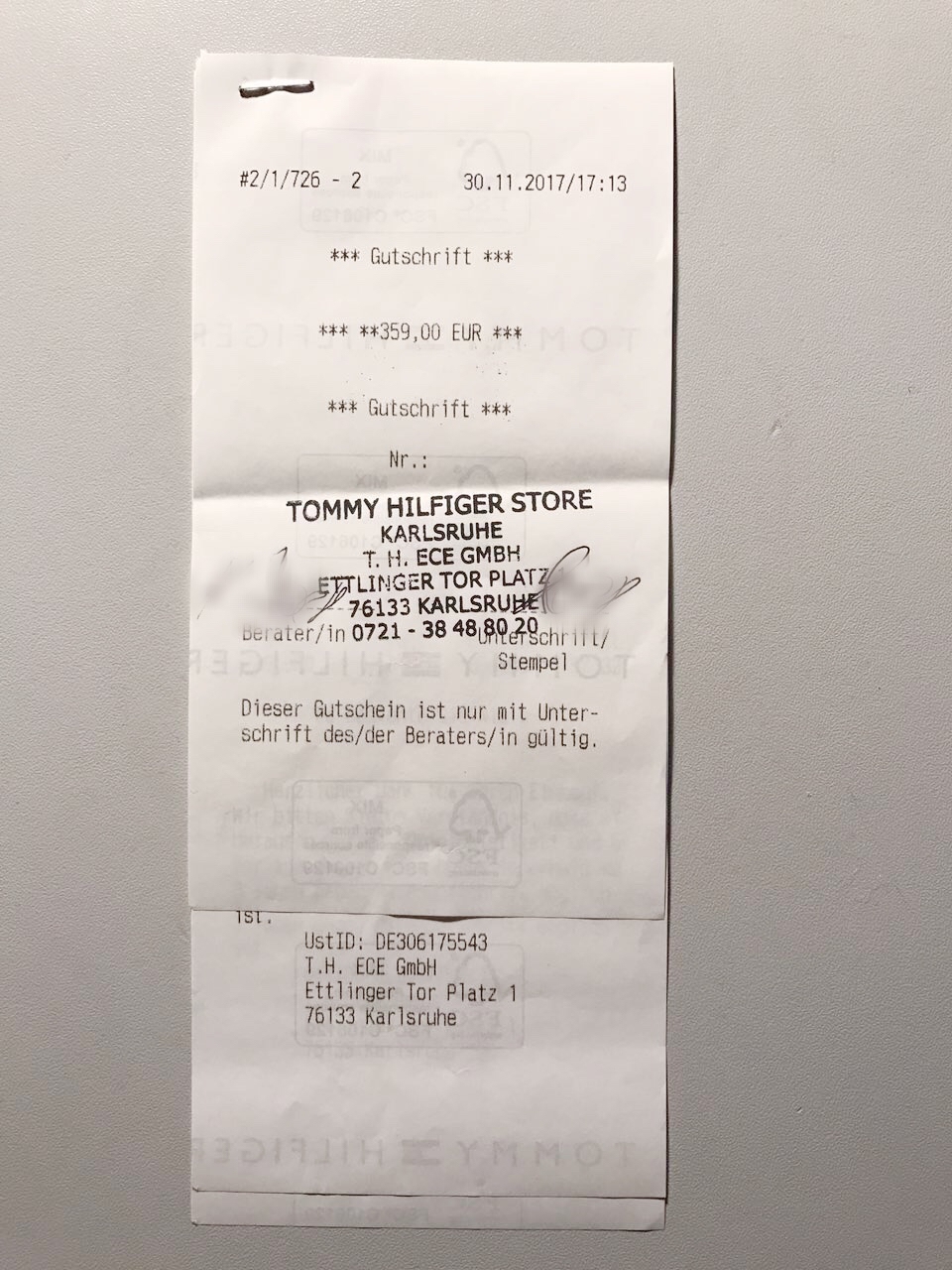The image depicts a close-up photograph of two thermal paper receipts, appearing to be stapled together at the top left corner, lying on a gray surface. The receipts bear signs of having been wet or digitally altered, particularly with some areas of blur or erasure. Key details can still be discerned:

- **Date and Time:** At the top right corner of the receipts, the date reads "30.11.2017" and the time "17:13" (5:13 PM).
- **Transaction Number:** On the top left, there is a series of numbers and symbols: "2-1/726-2".
- **Store Information:** There is an ink stamp, slightly askew, indicating it is from a Tommy Hilfiger Store in Karlsruhe: "Tommy Hilfiger Store, Karlsruhe, T.H.E.C.E.G.M.B.H., Ettlinger Tor Platz, 76133 Karlsruhe", along with a phone number: "0721-38488020".
- **Transaction Details:** The receipt prominently displays the word "Gutschrift" (German for "credit") with decorative stars around it, followed by the amount "359,00 EUR" (359 Euros), and then "Gutschrift" again.
- **Additional Information:** There's likely a store number denoted by "NR", followed by more German text, which could include terms related to the receipt being either a return or transaction receipt.

This detailed description compiles and emphasizes the repeating and shared elements across the given captions.